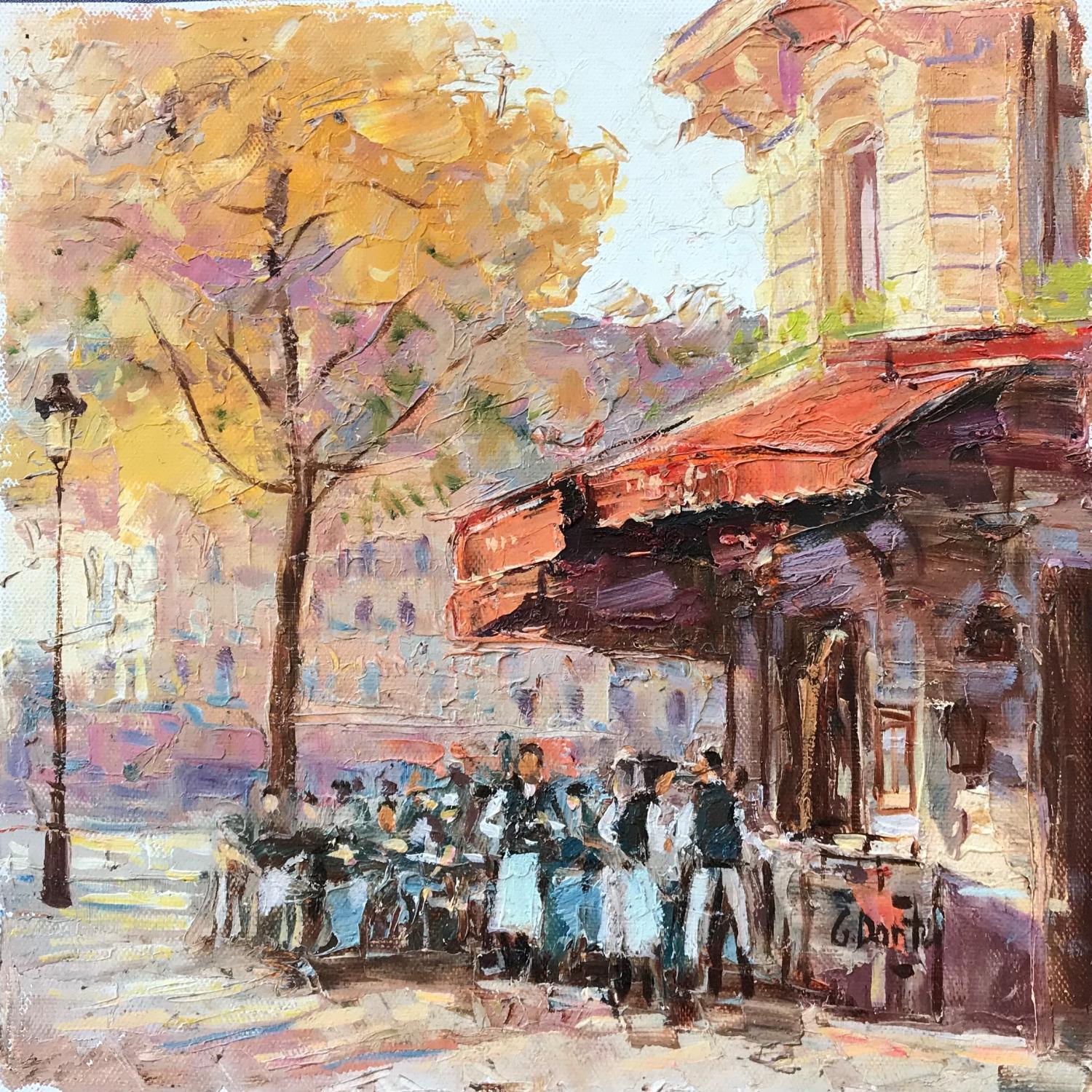This descriptive caption incorporates the shared and repeated details from each of the given accounts to create a detailed picture of the scene:

---

The oil painting, which appears impressionistic, depicts a bustling city scene, likely Paris, characterized by vibrant autumn colors. On the far left stands an old-fashioned black streetlamp next to a large tree with a textured brown trunk and leaves in hues of yellow, pink, and peach, suggesting the fall season. The painting captures a lively outdoor café under a red awning, with several tables occupied by people whose details are blurred, consistent with the impressionist style. Waiters and waitresses in black vests, white shirts, white aprons, and likely black pants are visible, attending to the patrons. The café building, on a street corner, is light beige, two stories tall, and features a prominent tower-like structure. The cobblestone or brick road adds to the quaint, nostalgic ambiance. The painting, signed in the bottom right corner by an artist with a name resembling “G. Dante” or “G. Ponto,” showcases detailed brush strokes and pastel shadows in blues, purples, and greens, enhancing the scenic depth and texture of this Parisian autumn day.

---

This detailed caption amalgamates the individual observations into a cohesive and vivid portrayal of the image.